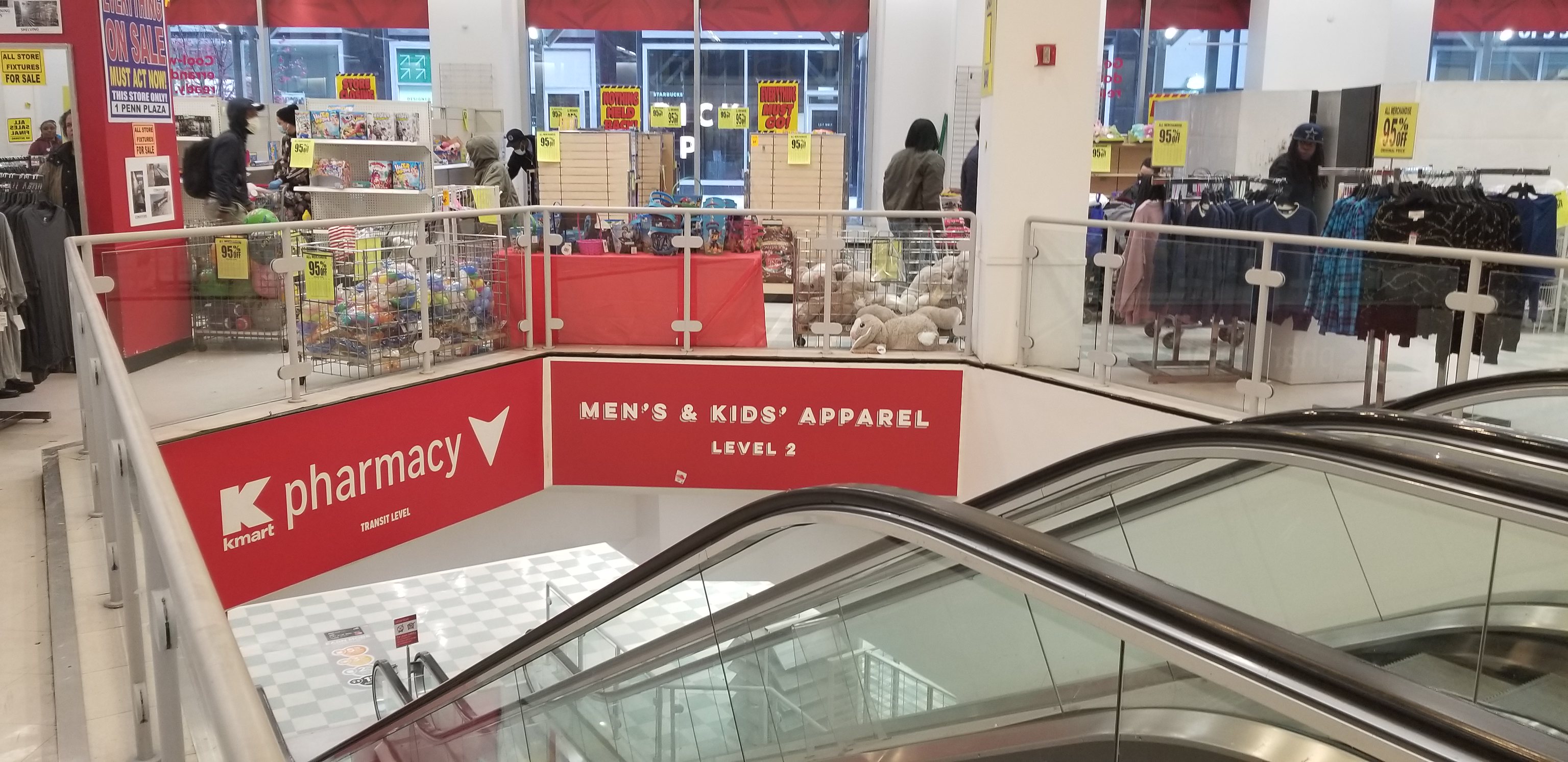This image captures a close-up view at the beginning of an escalator from the top. The escalator, devoid of any passengers, makes it unclear whether it ascends or descends. Parallel to this escalator is another, equally unoccupied. Directly across the way, a store specializing in children's merchandise is visible. Through several open entrances, you can spot colorful bins filled with bouncing balls and racks of child-sized clothing. Plush stuffed animals also pepper the scene. Prominently displayed in front of the escalator is a red sign that reads, "Men's and Kids Apparel, Level 2." Another red sign to the left bears the brand name "Kmart," accompanied by a white arrow pointing downward with the text "Pharmacy," indicating facilities on the first level.